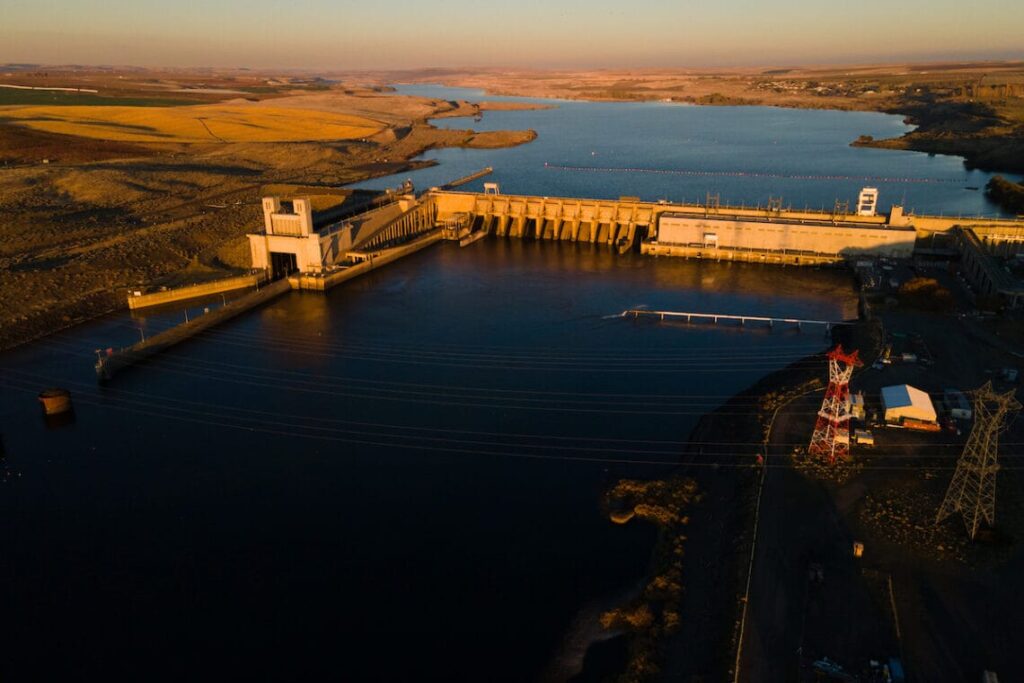The photograph appears to have been taken from a drone, showcasing an expansive and detailed aerial view of a large, deep blue waterway, likely a river managed by a concrete dam that also functions as a bridge. The scene is bathed in the atmospheric golden light of either sunrise or sunset, casting a warm hue over the landscape. The dam, featuring multiple sections that control water flow, is instrumental in preventing flooding of the surrounding regions.

The surrounding land on both sides of the river appears dry and barren with a yellowed or brownish hue, indicative of either the arid conditions or the specific time of day. On the right side, near the dam, there are intricate, spindly man-made structures, likely electrical towers, the most prominent of which is red and white. Adjacent to this tower stands a small building with a blue roof, white trim, and yellow siding, adding a splash of color to the otherwise muted environment.

In the background, the hazy, greenish-tinted sky further emphasizes the vastness and serenity of the scene, while to the left, a faint patch of green suggests an area irrigated by a visible pipe. Lastly, a modest dock extends into the river, enhancing the composition of this meticulously captured and descriptive aerial image.